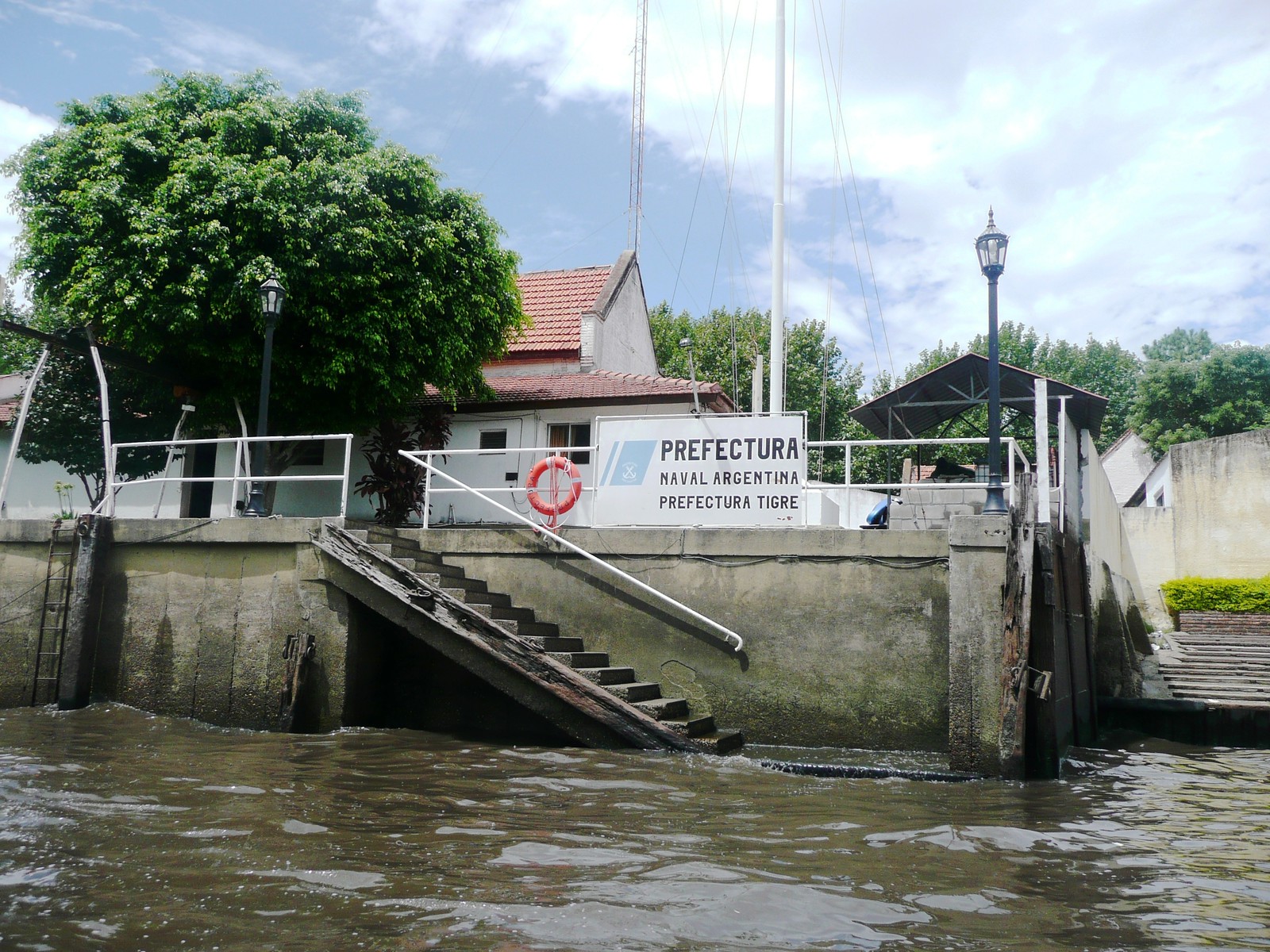The photograph captures a historic dock area in Tigre, Argentina, clearly marked by a sign that reads "Prefectura Naval Argentina Prefectura Tigre." Central to the image is a weathered dock with a low tide exposing moss-covered steps leading down to murky brown water. At the corner of the dock stands a lamppost on a cement base. Surrounding the dock are various structures: a metal pipe fence, stone walls higher than the water level, and a white building in the background. To the left, a tall green tree adds greenery against a backdrop of blue sky and white clouds. A life preserver ring hangs on a white railing descending the stair area, and there's a ladder on the left side allowing access to the water. The outdoor area prominently features concrete surfaces, with steps and platforms spanning down towards the water from the dock area.